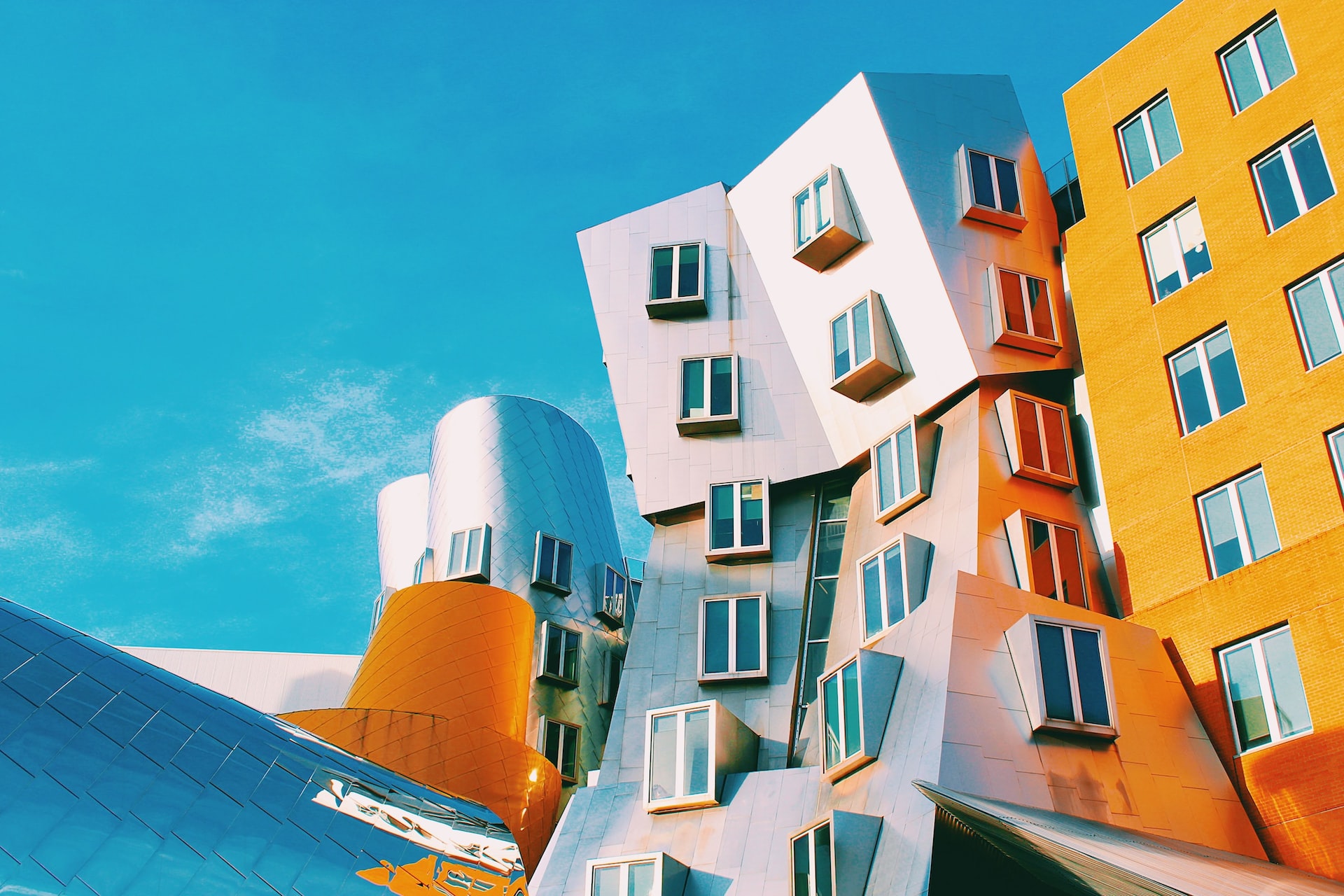This detailed, horizontally aligned, computer-generated image depicts the abstract representation of notable Cambridge architecture with a sense of disintegration. Dominated by a clear blue sky accented with feathery white clouds on the upper left side, the central focus is a series of buildings that appear to be falling apart. In the middle, a prominent white building spans at least six or seven stories, with its top two levels precariously tilting forward as though ready to collapse. Adjacent to it on the right is a yellow building of similar height, distinguished by its white-framed blue windows, standing more upright with only a slight leftward lean.

To the left of these central structures, there are two rounded buildings with windows, forming a cone shape at their base and leaning towards the left. Further left, a roundish building also features numerous windows. Below this structure is an element with an orange hue resembling the top of a detergent cap. The lower left corner reveals a shiny blue-gray rooftop with visible shingles, adding to the collage of architectural forms. Overall, the image integrates traditional and abstract elements, making the buildings seem both recognizable and artistically distorted.